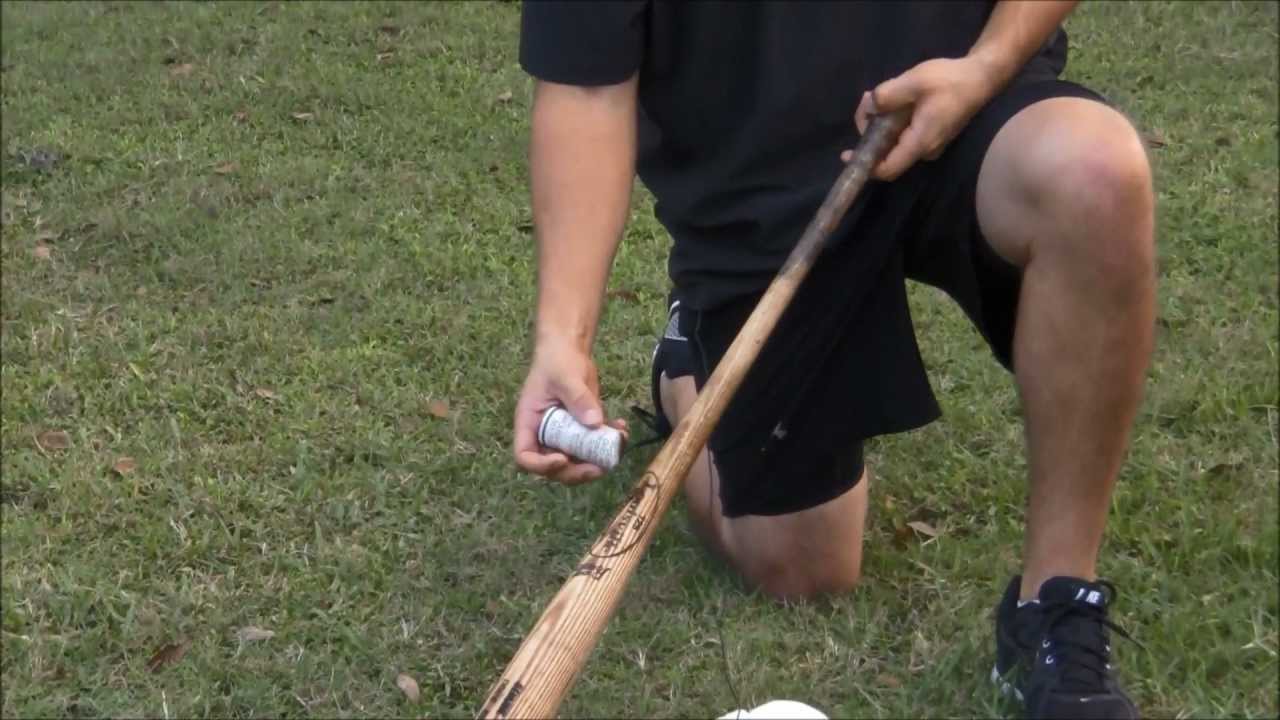This image captures a Caucasian man, viewed from the shoulders down, kneeling on a grassy green lawn in the afternoon light. He is dressed in a black t-shirt with elbow-length sleeves, black shorts, and black tennis shoes. The man is in a crouching position, with his right knee on the ground and his left leg bent to support him. In his left hand, he holds a tan-colored wooden baseball bat, which darkens towards the end he is gripping. The bat features a brown circle with brown lettering. In his right hand, he is holding a white object, possibly a stick with a brown tip, which might be paint or varnish. It seems he is either painting or repairing the bat. The grassy background completes the outdoor setting.